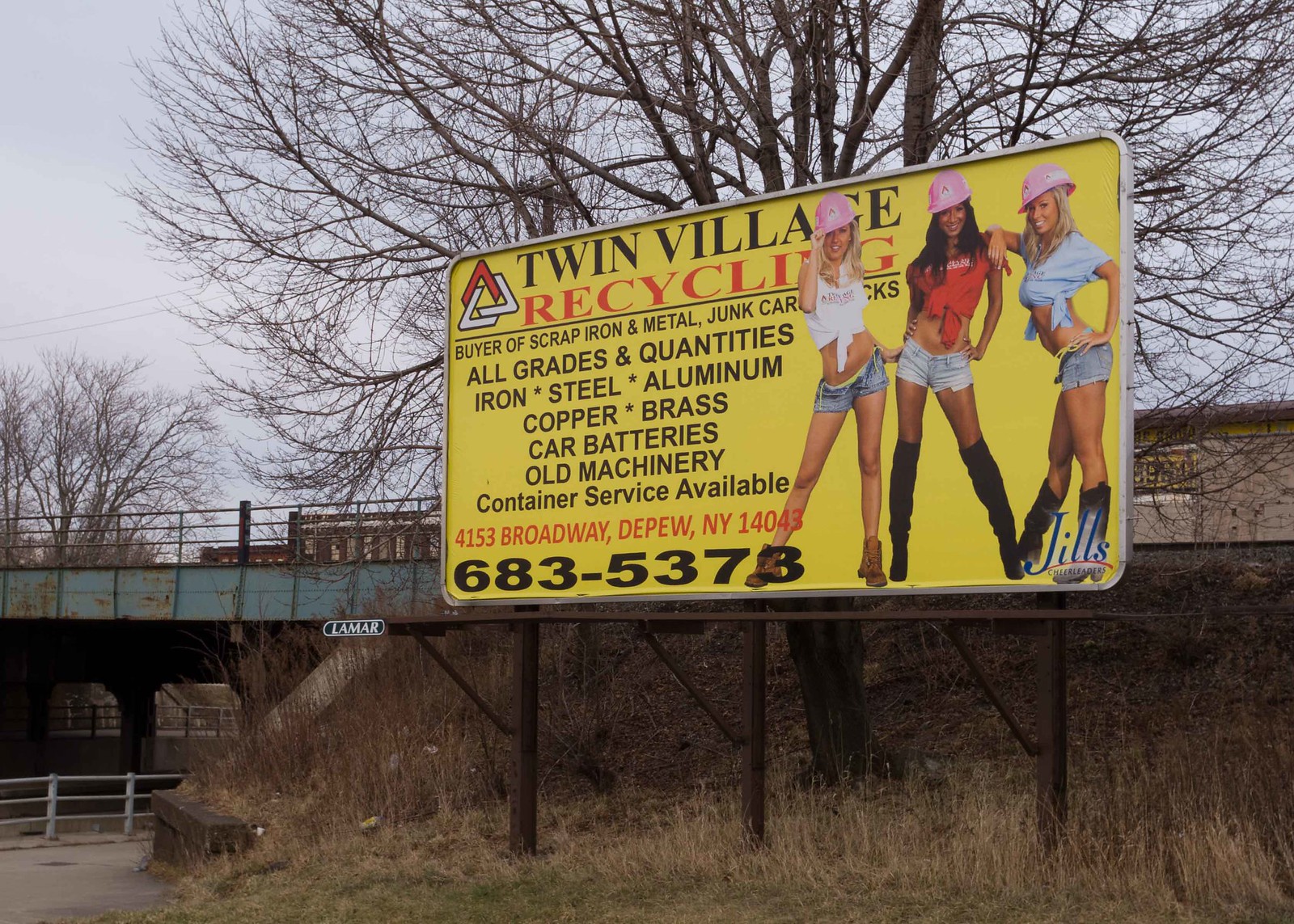The image captures an outdoor billboard positioned next to a rusty, old railroad bridge or overpass. The scene it is set in is late fall or winter, featuring a barren tree with no leaves and overgrown, brownish grass. The bright yellow billboard, supported by three posts with a dark walkway, advertises Twin Village Recycling, a buyer of scrap iron, metal, junk cars, and trucks. The billboard displays the company’s services in buying all grades and quantities of iron, steel, aluminum, copper, brass, car batteries, and old machinery, with container service available. It provides the address, 4153 Broadway, Depew, New York 14043, and phone number, 683-5373. On the right-hand side of the billboard, three scantily dressed Caucasian women in suggestive poses are wearing pink hard hats, midriff tops, short denim shorts, and a variety of brown and black boots. The name "Jill's" is mentioned on the bottom right corner of the billboard. The company's logo, consisting of three intertwined triangles, one of which is red, is also present.